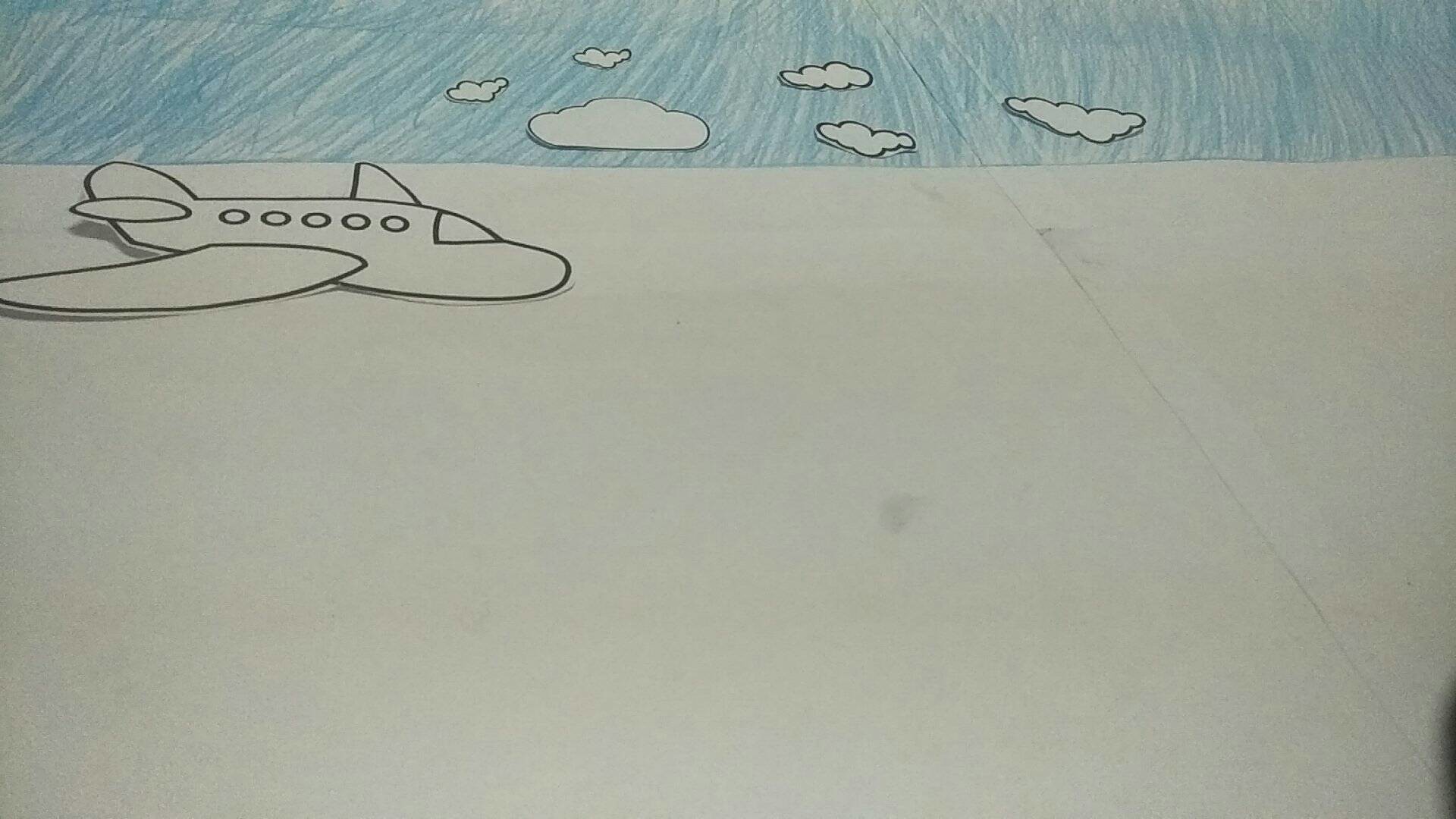The illustration presents an imaginative, collage-style depiction of an airplane soaring through a slightly whimsical sky. The background is a serene, light blue, filled with fluffy, white clouds that appear to have been intricately cut out and pasted onto the paper, creating a sense of depth. Adding to the collage effect, the airplane itself seems like a cutout, meticulously placed in the scene. The aircraft features a single wing, five windows along its side, a prominent tail at the back, and a detailed cockpit with a window at the front, suggesting that it is in-flight. Notably, a strip resembling tape runs diagonally from the middle towards the upper-right corner, which adds an element of texture to the composition. The paper shows subtle smudge marks, lending a slightly imperfect and handcrafted feel to the artwork.